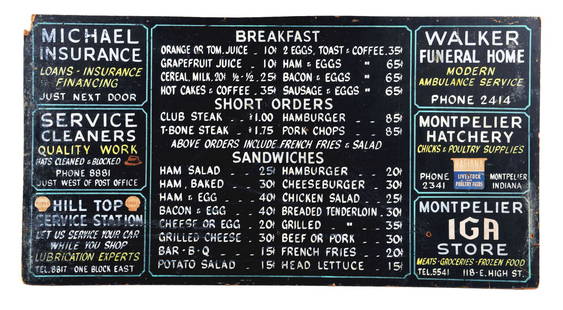This image portrays a vintage menu board, likely from the early 1900s, featuring a variety of advertisements for local businesses. The board itself is black with white acrylic paint marker writing and minimal, straightforward designs, such as a hat and symbols, with a small banner indicating the businesses. The central portion of the board displays a simple menu divided into categories: breakfast, short orders, and sandwiches. Breakfast options include items like orange or tomato juice for $0.10, hotcakes and coffee, and various egg dishes, with prices reflecting the era's affordability, such as bacon and eggs for $0.65. Short orders list club steak, t-bone steak, hamburger, and pork chops, each accompanied by french fries and salad. Sandwiches include ham salad, grilled cheese, barbecue, hamburger, and chicken salad, with add-ons like french fries and head lettuce.

Flanking the menu are six distinct advertisements for local businesses: 
1. Michael Insurance: Loan insurance financing, located next door.
2. Service Cleaners: Quality work on hats, just west of the post office.
3. Hilltop Service Station: Car servicing while you shop, lubrication experts, one block east.
4. Walker Funeral Home: Modern ambulance service, phone number 2414.
5. Montpelier Hatchery: Chicks and poultry supplies, based in Montpelier, Indiana, featuring a shield logo.
6. Montpelier IGA Store: Meats, groceries, frozen foods, located at 118 East High Street.

The combination of the central menu and side advertisements, along with the period-specific pricing and services, offers a glimpse into the local commerce and dining options of the time.